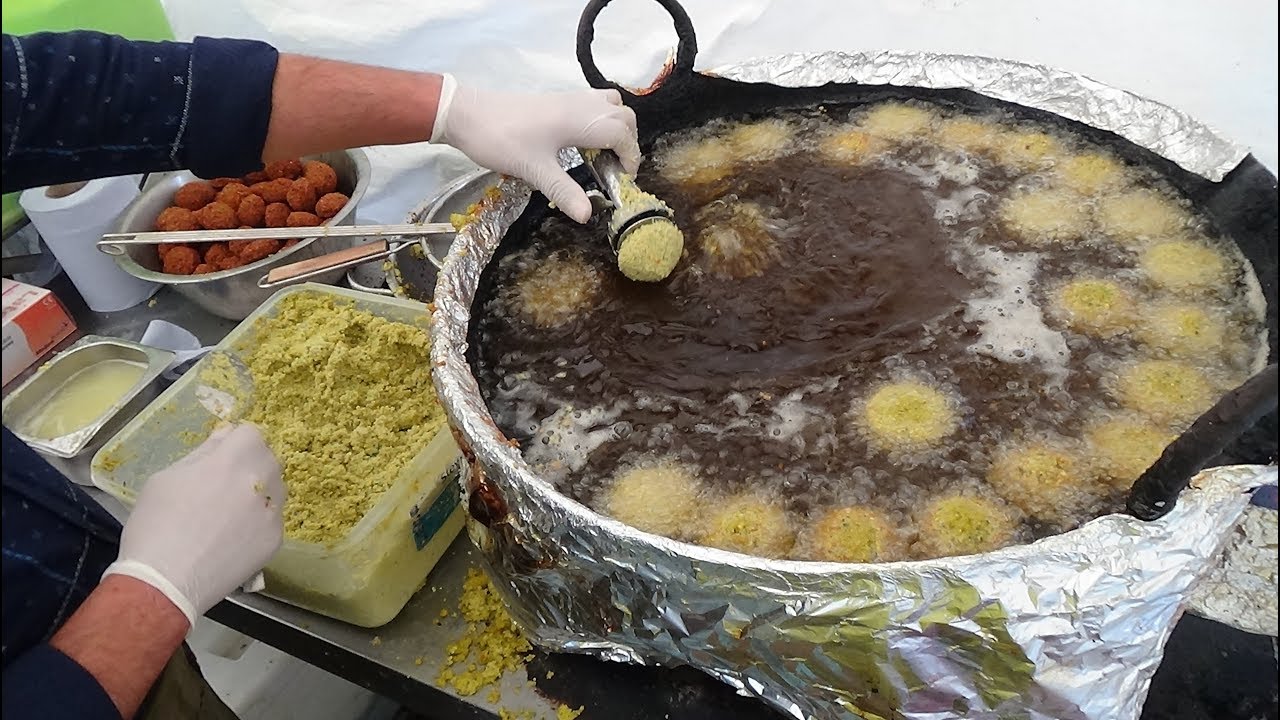In this photograph, a man, dressed in a blue shirt with rolled sleeves and wearing white latex gloves, is preparing food over a large, cast-iron pot filled with bubbling hot oil. The pot, which does not have a lid, has aluminum foil wrapped around its edges. The man is using a silver-colored scoop to drop a granular yellow-green substance, possibly grated cheese or dough, into the oil. His other hand is reaching into a large plastic container filled with this substance, preparing to add more to the pot. The pot already contains around twenty small, ball-shaped pieces floating in the oil. Additionally, there is a spoon and stainless steel bowls holding a yellow-green paste nearby. A roll of paper towel and a container with more latex gloves can also be seen on the floor on the left side of the image, indicating this is a professional or well-organized kitchen space.